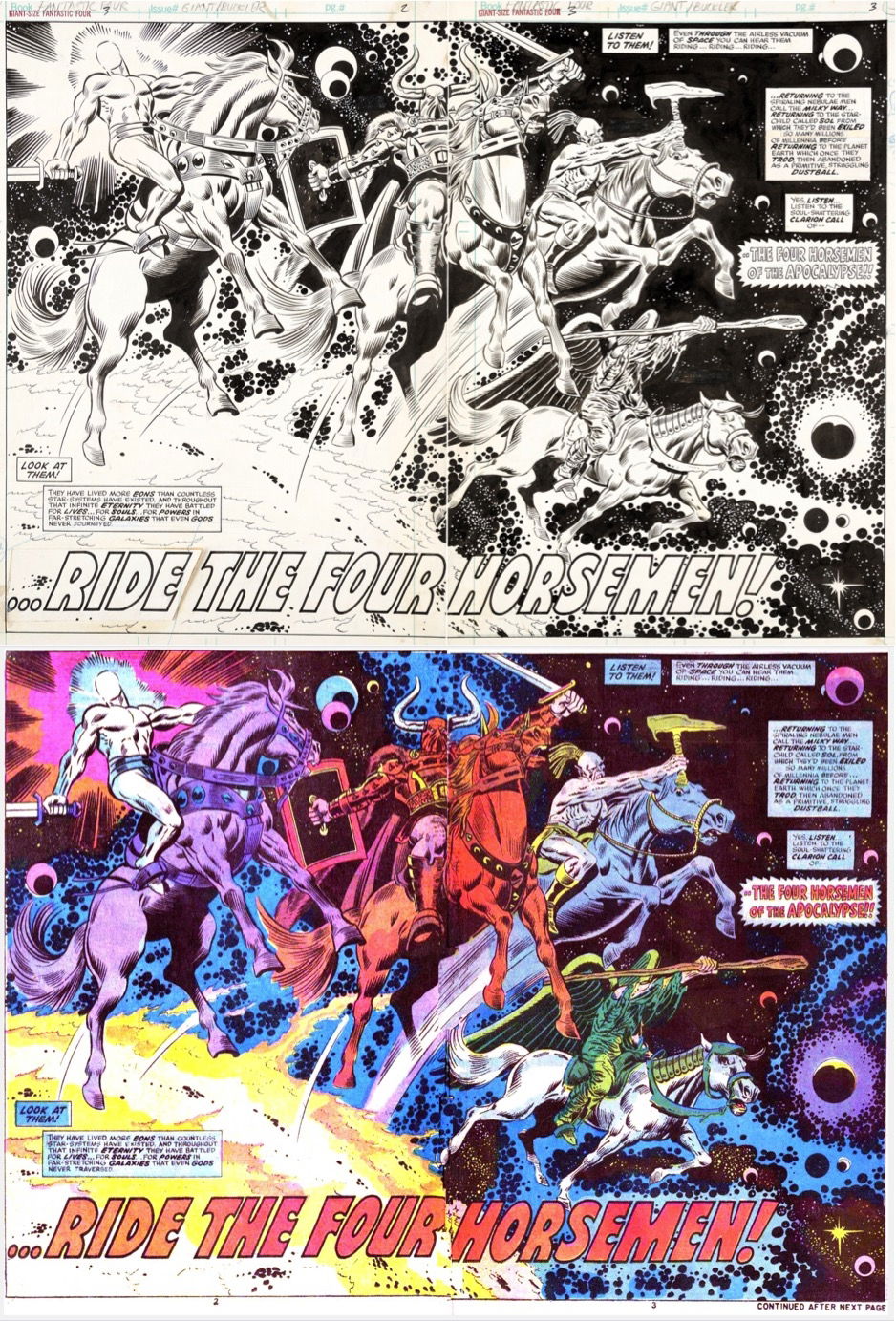The image is divided into two vertically stacked comic book panels, with the top panel in black and white and the bottom panel in vibrant color. Both panels depict the same dynamic scene of four imposing figures riding through space, each on a distinctively colored horse. The vibrant colors highlight a shiny being on a purple horse, a horned villain on a red horse, a helmeted individual on a blue horse, and a green-winged figure holding a staff on a white horse. These figures evoke the imagery of the Four Horsemen of the Apocalypse. The bottom image features bright costumes matching the horses, including a green-costumed figure with wings and a shield-bearing character in red. Both images contain the bold words "Ride the Four Horsemen" in large white letters outlined in black, emphasizing their formidable presence.